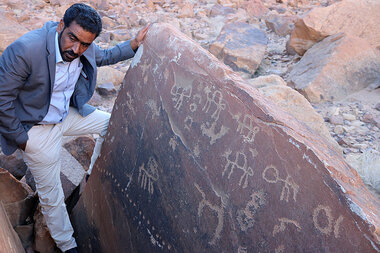In this somewhat grainy, square image, a Middle Eastern man with dark hair, a moustache, and a beard stands amidst a large pile of rocks, gazing slightly downward to his right. He is dressed neatly in light khaki pants, a light blue button-up shirt, and a light blue jacket, layered under a darker blue or grayish-blue dress jacket. His hand rests on an ancient, massive stone slab measuring around 10 by 8 feet, which is covered in intricate inscriptions or carvings that resemble ancient scribbles or symbols, potentially thousands of years old. The background consists of more rocks, suggesting the photo was taken in an outdoor setting resembling a quarry or an archaeological site, and the overall image has a nostalgic, slightly blurred quality as if it were taken in the 1980s.